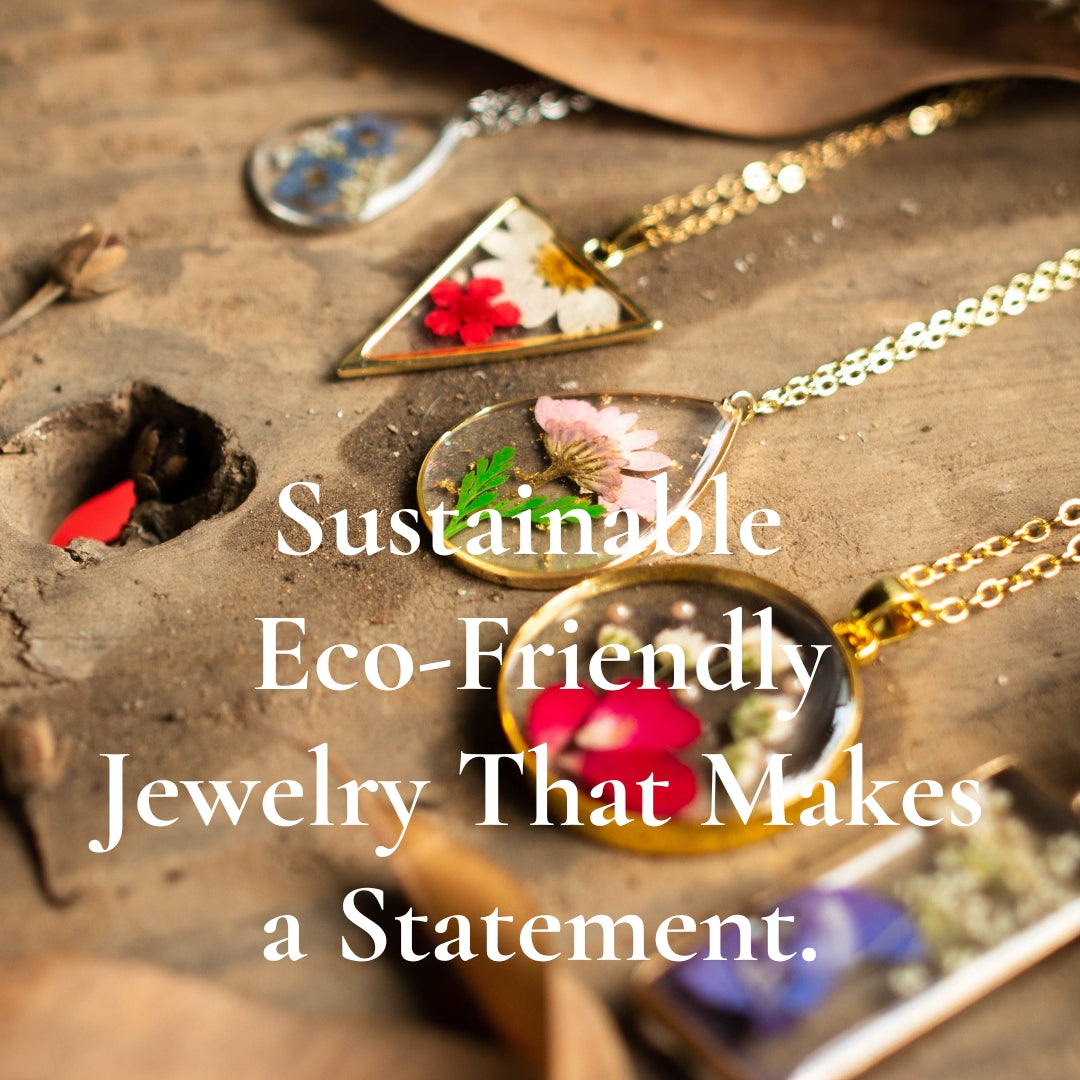This is a detailed depiction of an advertisement for a jewelry brand showcasing five unique necklaces laid out against a rough, earthy stone background. The necklaces are arranged vertically, with their chains extending to the right side of the image, creating a natural flow. 

1. **Top Necklace:** A silver piece featuring delicate blue flowers, though they’re somewhat faint.
2. **Second Necklace:** A gold triangular pendant with a pressed arrangement of white and red flowers encased in glass.
3. **Third Necklace:** A gold teardrop pendant containing a vibrant pink flower accompanied by green leaves.
4. **Fourth Necklace:** Another gold piece, this one circular, embedding white flowers and a striking red flower.
5. **Bottom Necklace:** The final piece, either gold or rose gold, slightly blurred, encasing a purple flower.

Over the necklaces, the text reads: "Sustainable, eco-friendly jewelry that makes a statement," emphasizing the brand's commitment to environmental consciousness while highlighting the intricate beauty of the pressed flowers in each unique piece.